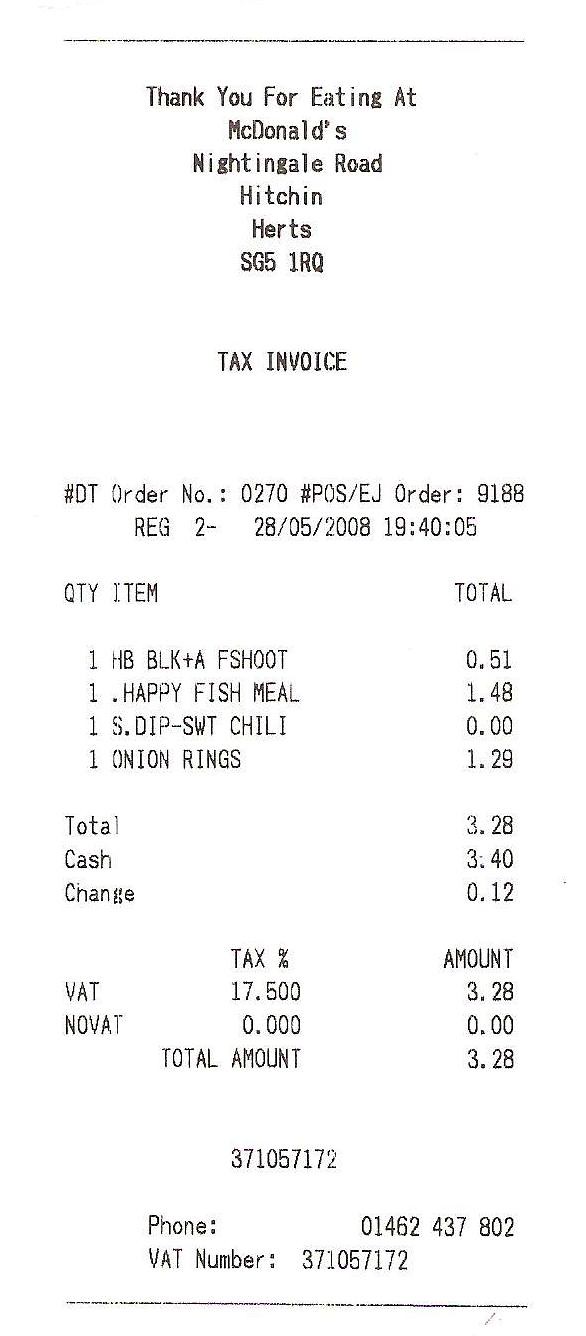This image showcases a McDonald's receipt from the Nightingale Road location in Hitchin Hurt, with the postal code SG5 1RQ. The receipt, printed in black text on a white background, begins with a "Thank you for eating at McDonald's" statement at the top. There are black horizontal lines framing the top and bottom of the receipt. Below the heading, it states "Tax Invoice" followed by several numbers and codes: "DT," "Order Number 0270," "POS/EJ Order 9188," "REG2," and a series of numerical codes including "2805," "2008," "1940," and "05."

The main section of the receipt lists the purchased items and their quantities. On the right-hand side, each item is matched with a corresponding total. At the bottom, the receipt concludes with a breakdown of the total charges, specifying the payment method with "Total Cash Charge." Additionally, the receipt includes the contact phone number "01462 437802" and a VAT number "371057172." The overall formatting is neat and structured, with clearly defined sections for easy reading.